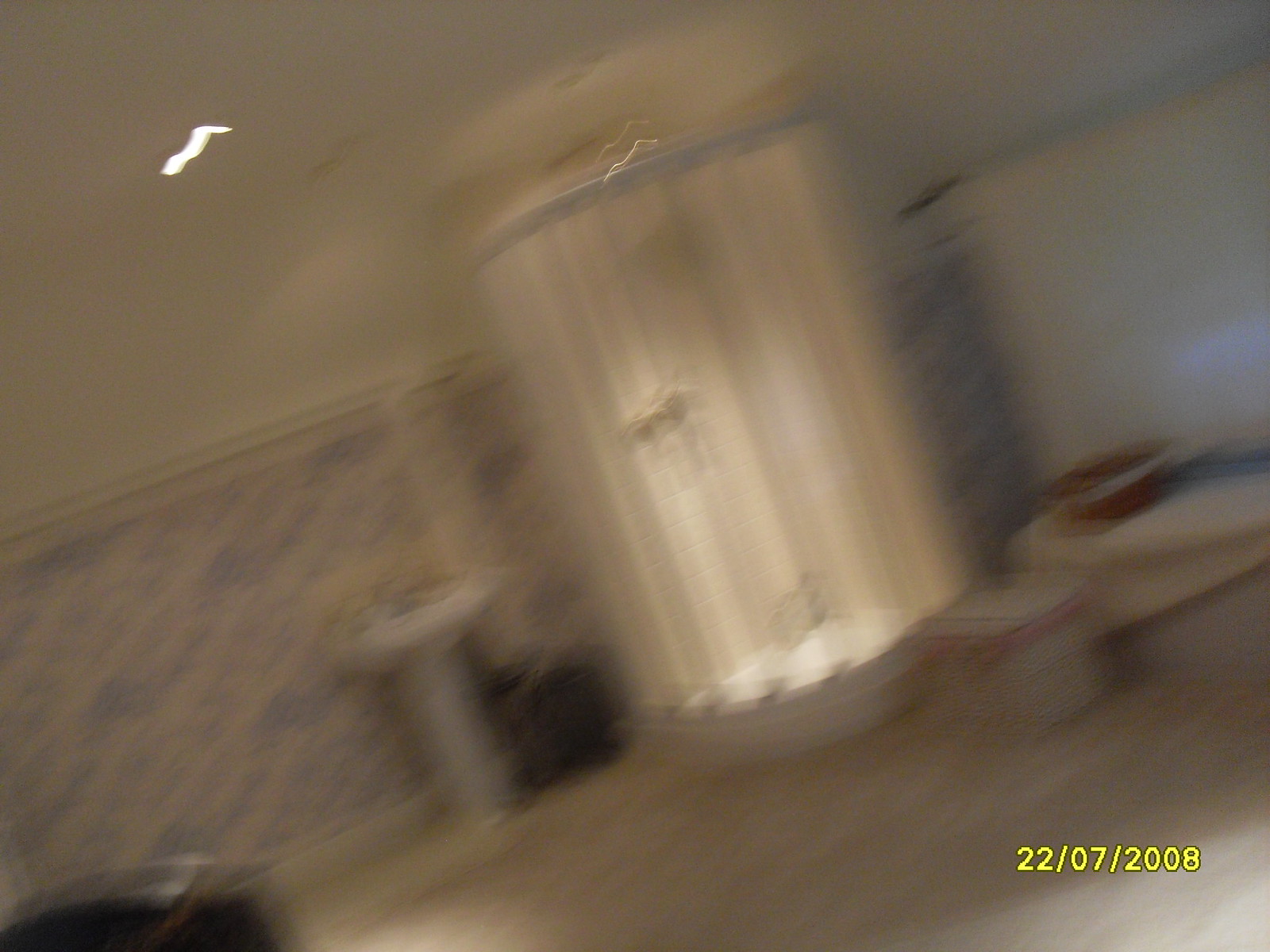A hazy, blurry horizontal photograph captures the interior of a spacious, modern bathroom. The main focus is a contemporary quarter-circle enclosed shower, illuminated from within. To the left of the shower stands a pedestal sink adorned with elegant gold fixtures. To the right, a bathtub with a tray poised over it is adjacent to a bench, with a closed curtain partially visible. The walls feature a blue and white patterned wallpaper, while the floor is a blend of white and beige hues. The ceiling is white, reflecting the shower's light. In the bottom right corner, the yellow date stamp reads "7-22-2008."